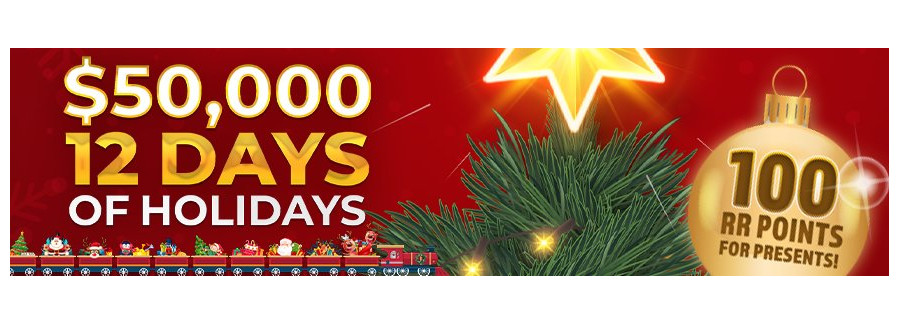The image is a festive holiday-themed rectangle with a predominantly red background. Upon closer inspection of the left side, the red backdrop is enhanced with subtle floral patterns and linear designs that resemble Christmas tree leaves. 

In the upper left-hand corner, prominently displayed, is a white text with a gold border that reads "$50,000." Directly beneath it, in a striking goldish-yellow hue, the text "12 DAYS" appears in bold, all-uppercase letters. Following this, the words "OF HOLIDAYS" are also in bold, full-capital letters, but in white.

To the right, the top section of the image features a radiant golden-yellow star, complete with illustrative shining glares, mimicking the effect of a star atop a Christmas tree. Below this star, there are two decorative lights.

Moving to the upper right-hand corner, there's an ornate bell-shaped design in gold and brown hues, which reads "100 R points for presents." Additionally, the lower section of the image depicts a cheerful Christmas scene with a detailed red train adorned with gifts, a Santa Claus figure, and miniature Christmas trees.